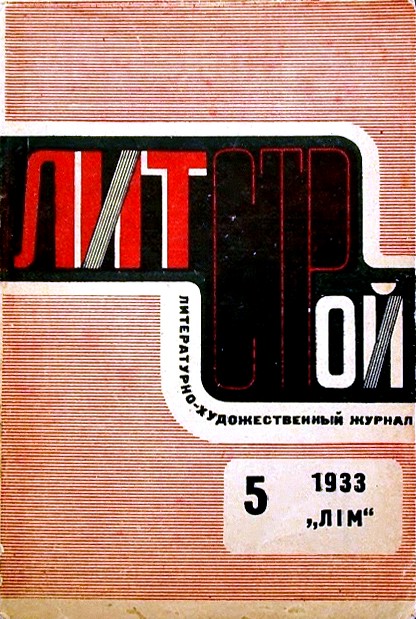The image appears to be a vintage-style poster from Eastern Europe, likely from the Soviet Union era. The background features red and white horizontal stripes, giving it an old-fashioned look. Dominating the center of the poster is a company logo composed of red, black, and white colors, featuring foreign characters, likely Cyrillic, suggesting Russian origin. In the lower right corner, the number "5" stands out prominently against a white imprint, along with the year "1933" and what appear to be Cyrillic letters underneath. Additionally, there are complex arrangements of letters and patterns running across the stripes, with some letters bordered in white and others on a black background. The arrangement forms intricate paths, resembling a pipe juncture with letters such as N, X, T, C, P, and O. Despite the language barrier, the poster's vintage aesthetic and the detailed yet cryptic lettering suggest it could have been a promotional or informational poster from that historical period.